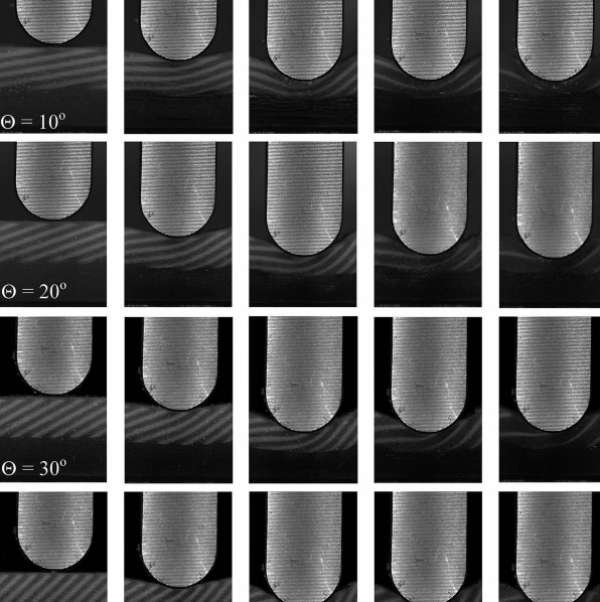The detailed image consists of four rows of five black-and-white, rectangular microscopic photos each, forming a grid. Each row documents a process where a gray, U-shaped object gradually pushes into a line or bar resembling wood, depicted in a cross-section manner. In the first row, labeled with "equals 10 degrees," the sequence begins with the U-shaped object barely touching the bar. Successive images show the object pushing deeper, causing slight indentations that progressively deepen until the object is almost fully embedded in the final picture. The second row, labeled "equals 20 degrees," mirrors this process, but with the U-shaped object pressing even deeper into the bar. The third row, labeled "equals 30 degrees," follows the same pattern with even more pronounced indentation. The fourth row, although the label is cut off and presumed to be "equals 40 degrees," demonstrates the deepest penetration yet, with the U-shaped object significantly distorting the bar. Throughout the sequences, the background remains a stark black, accentuating the changes in the bar's shape and the intricate details of the indentation process.